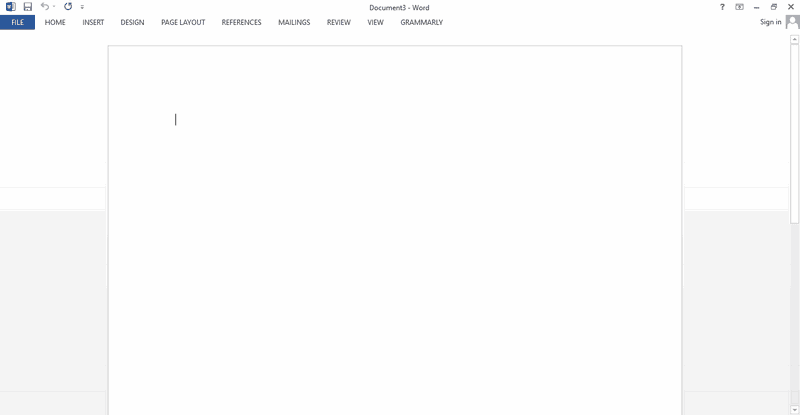This image is a screenshot of a computer screen with a horizontally rectangular shape. The background is divided into two sections: the top half is white, and the bottom half is light gray. Dominating the center of the screen is a large white square, outlined with a light gray line on three sides, leaving the bottom edge open. Inside this square, there is a horizontal gray line on the left side, positioned about five lines down from the top, resembling a cursor. On the right edge of the screen, there is a vertical scroll bar. In the upper left corner of the screen, a few indistinct icons are visible. Below these icons, there is a menu bar that includes options such as File, Home, Design, Page Layout, References, Mailings, Review, View, and Grammarly. The "File" menu option, located on the far left, is highlighted with a blue rectangle. At the very top center of the screen, the document title is displayed in gray text within brackets, followed by the word "document - Word."